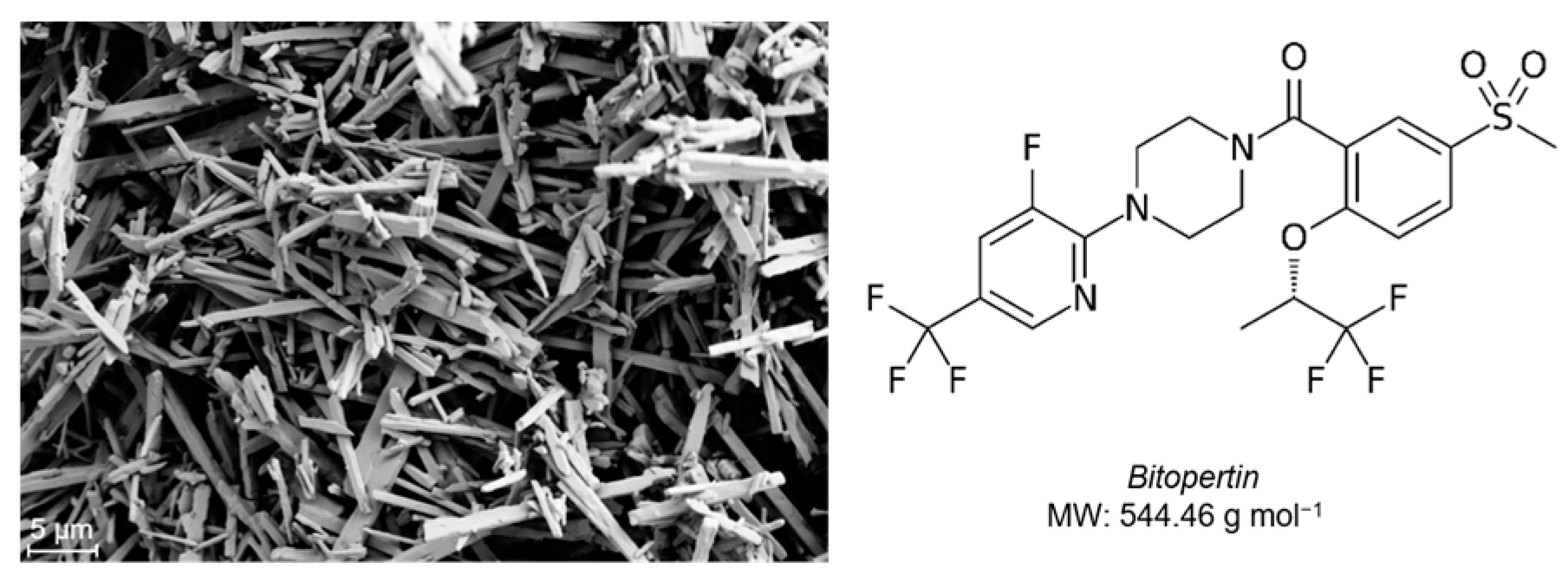This rectangular image, approximately five inches wide and two inches high, is divided into two distinct sections. On the left side, there is a black and white, up-close microscopic photograph displaying a network of interconnected fibers or stick-like structures, appearing in varying shades of gray. The background is a solid black, highlighting these intricate, tangled forms. In the bottom left corner, white text indicates the measurement "5μm" (micrometers).

On the right side of the image, set against a plain white background, there's a detailed molecular structure. This structure consists of hexagonal (honeycomb) shapes interconnected with lines, representing chemical bonds, and includes the elements F (Fluorine), N (Nitrogen), O (Oxygen), and S (Sulfur). Above this molecular diagram, in bold black print, is the name "BITOPERTIN." Below the structure, the text reads "MW 544.46 G/MOL."

This dual-image presentation showcases, on the left, an intricate view of a fibrous material at the microscopic level, and on the right, the molecular configuration of a compound named BITOPERTIN.